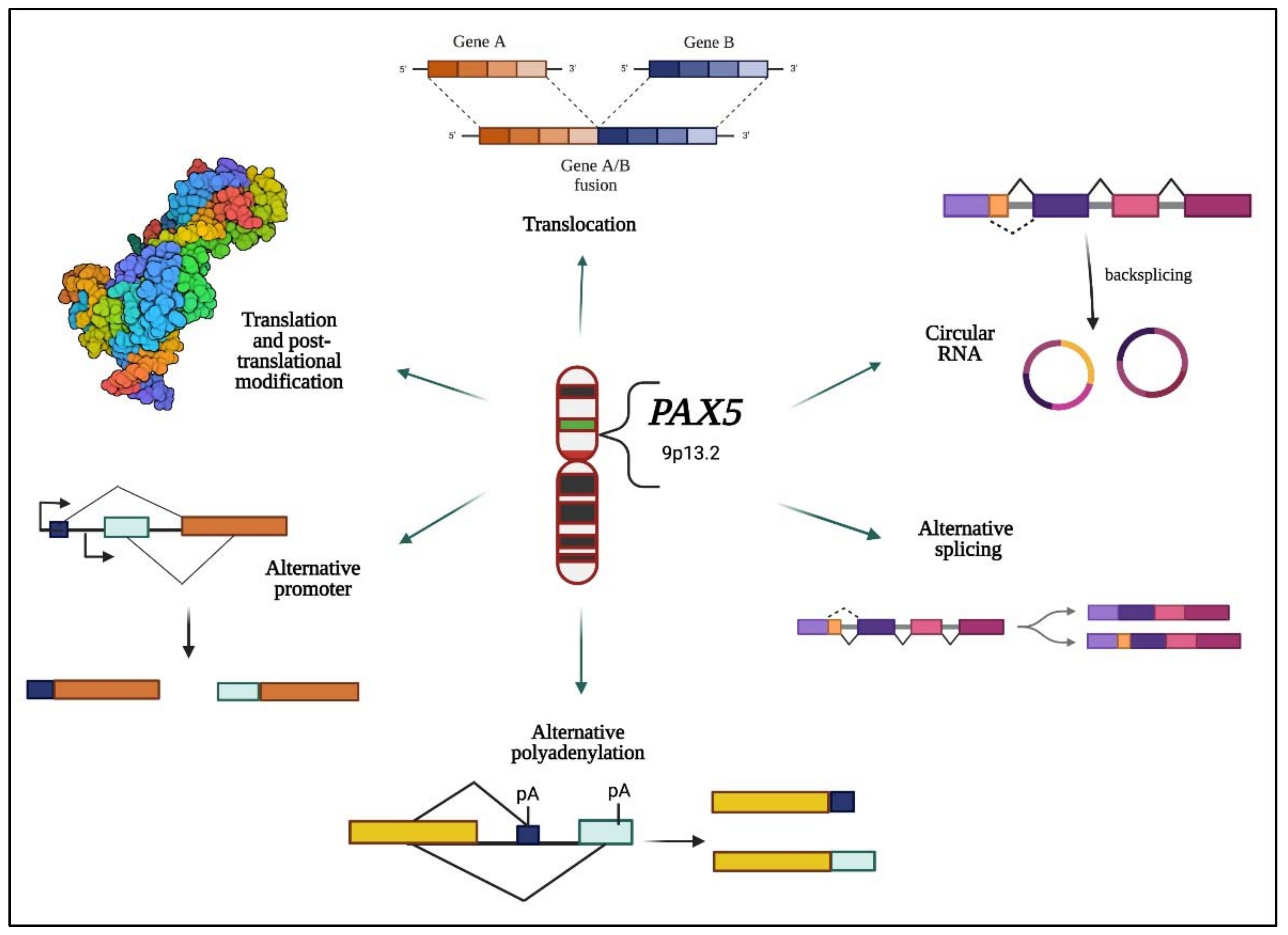This detailed scientific illustration and flowchart presents a comprehensive overview of various genetic operations through a series of colorful, intricate diagrams. Dominating the center of the image are two pill-shaped genetic cell representations labeled PAX5 and 9P13.2, from which arrows radiate in six different directions, each leading to specific genetic processes. At the top, an arrow points to "translocation," illustrating the fusion of gene A and gene B. To the left, the top label reads "translation and post-translational modification," represented by a multicolored blob, and beneath it, "alternative promoter." The bottom of the illustration points to "alternative polyadenylation," showcasing numerous colorful rectangles and squares. On the right-hand side, the upper label points to "circular RNA" next to "back splicing," while below is "alternative splicing," again accompanied by a multitude of colorful bars in shades of yellow, light blue, purple, dark purple, pink, and orange. The use of diverse shapes and vibrant colors vividly captures the complex interactions and modifications in genetic processes, making it a detailed and educational depiction of genetic operations.